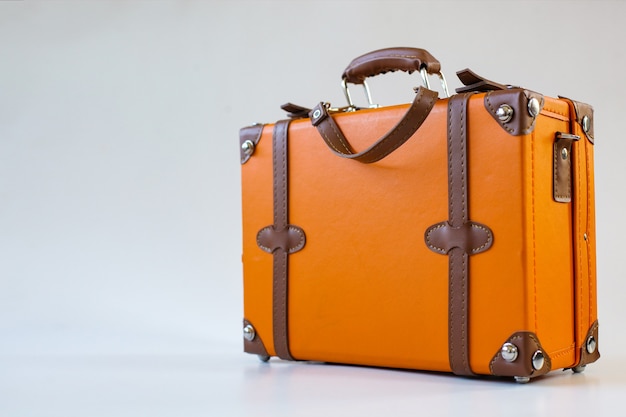This image showcases an orange suitcase with brown leather accents, standing prominently against a white background. The suitcase occupies much of the frame, dominating the space from the middle to the right edge and from top to bottom, while the left side remains as blank white space. The suitcase features brown leather straps on its front, as well as brown leather patches on its corners, which are fixed in place with small silver screws or buttons. Additionally, it has a sturdy brown handle attached to the top via two little metal pieces. The overall design appears durable and spacious, suggesting that it can accommodate a considerable amount of clothes. The clean, minimalist background places all attention on the unique and distinctively styled suitcase.